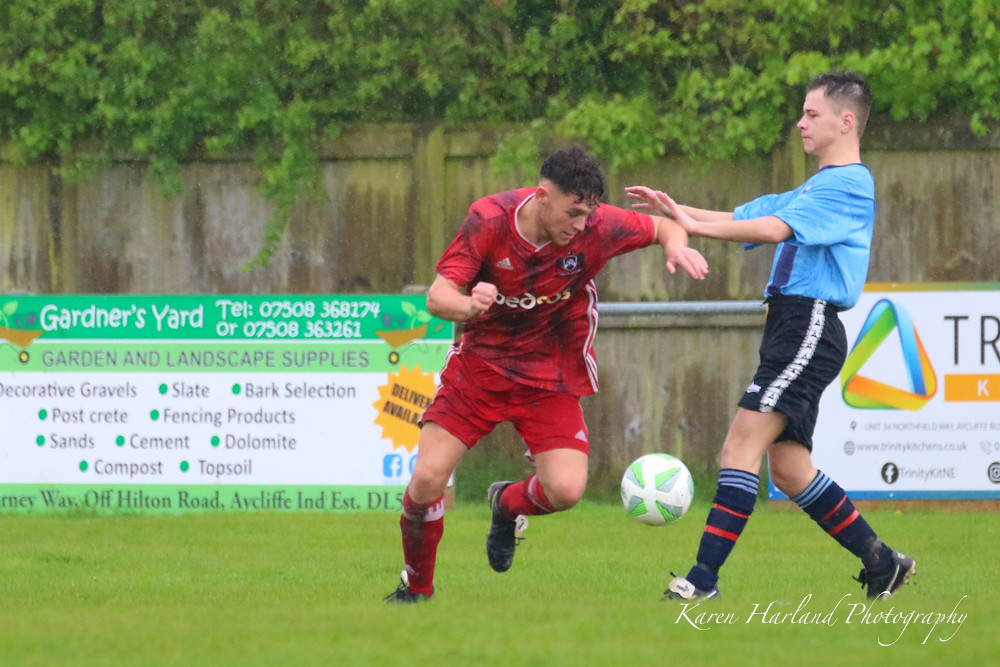In this horizontally aligned rectangular picture, two men are captured on a grassy soccer field, positioned centrally in the frame. The man on the left is in mid-action, preparing to kick a white and green ball that is suspended in the air. He is dressed in red shorts and a red jersey that features some white stripes down the side and an Adidas logo on his chest, although the other print is unreadable. He has a distinctive hairstyle with shaved sides above his ears and longer, curly dark brown or black hair on top. 

To his right, another man appears to be attempting to block or push the first man, with his arms extended forward. This man is wearing a light blue shirt with black shorts, complemented by black and red socks. His hairstyle includes shaved sides with very short brown hair on top. 

The background reveals a wooden fence with trees hanging over it, along with a second, shorter wooden fence in front that has a metal railing. Prominent advertisements are visible on the fence: one reads "Gardener's Yard" and details garden and landscape supplies, while the other has a colorful triangular logo and the partial text "TR," cut off by the edge of the picture. In the lower right-hand corner, the photographer's watermark "Karen Harland Photography and Wildlife" is displayed.